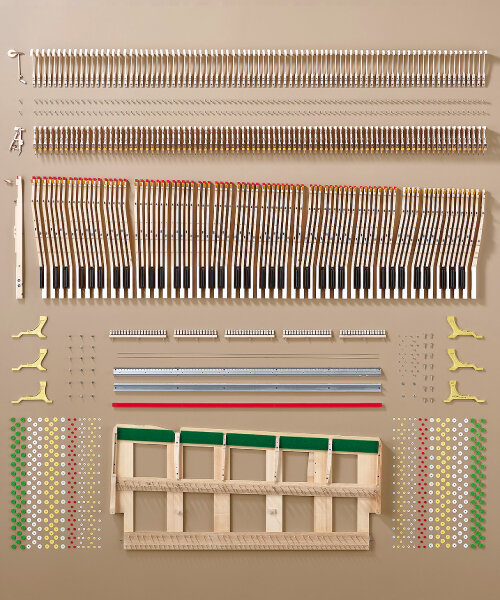The image displays a meticulously organized, disassembled assembly possibly from a musical instrument or an electronic device. The overall composition is rectangular with a beige background. At the very top, there is a row of small, uniform, white objects resembling q-tips, closely packed in a horizontal line extending across the image. Below this is a series of tiny cylindrical components in shades of white, brown, and gold. Directly beneath these are elongated, white pieces resembling keyboard keys, suggesting they might be parts of a piano mechanism or serve a similar function. Further down, there are various multi-colored components—yellow, green, red, and gold—that are more substantially sized. Among these, there is a distinctive piece with a bent structure and a red top at one end. Near the lower part of the image, several smaller gold pieces and lines of screws, along with clusters of colored dots in green, white, gold, and red, are visible. Finally, at the very bottom, there is a large, angled wooden piece with green fabric at the top and multiple square cut-outs, indicating it may be a structural or supportive part of the entire assembly.